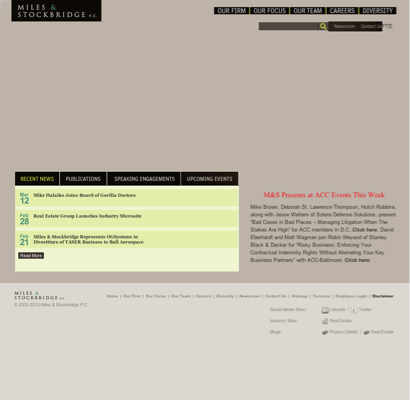This screenshot captures the home page of a website featuring a notably outdated design characterized by its simplicity and lack of images. The background is predominantly a large beige color, giving the site a very plain appearance. In the top left corner, there is a black box containing the company logo, which reads "Miles at Stockbridge" in white text, with the final symbol in green. 

The top right corner of the screenshot displays five black boxes, each containing a menu option: "Our Firm," "Our Focus," "Our Team," "Careers," and "Diversity." The lower half of the website transitions into a lighter beige color, encompassing the bottom third of the page. Positioned centrally within this lighter section, on the right side, is a passage of text. The screenshot is quite small, adding to the challenges of clearly seeing finer details. 

Overall, this minimalistic and rather dated design emphasizes basic navigation while lacking modern visual elements and imagery.